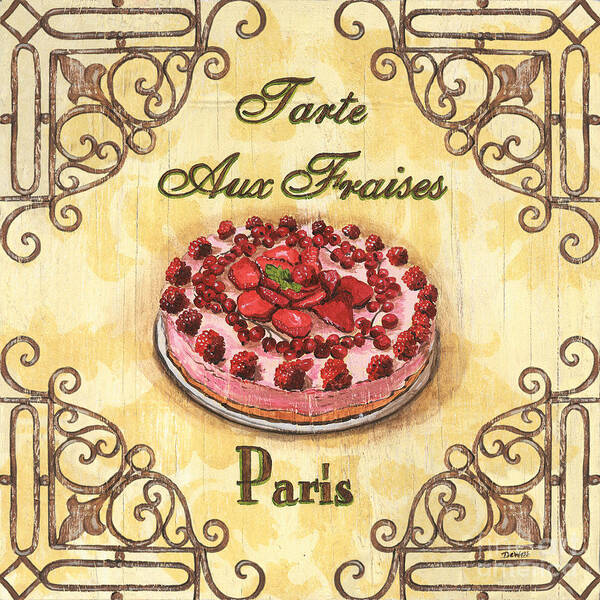The image seems to be an artistic depiction, likely designed as a cover or sign, inspired by French aesthetics. It features a central illustration of a vibrant and colorful strawberry tart, possibly accompanied by raspberries and cherries, rendered in a drawing or animated style rather than a real photograph. The tart sits on a serving dish against a light brown, beige, and creamy yellow background, giving a rich, buttery impression with hints of autumnal tones. Intricate, filigree metal work designs embellish each corner, incorporating fleur-de-lis motifs, lending a classic French elegance reminiscent of wrought iron railings or grates. The top of the image displays the text "Tarte à la Française," and the word "Paris" is written beneath the tart in brown text with a green outline. This detailed and decorative piece could serve as a sign for a Parisian pastry shop, a cover for a restaurant menu, or an art piece for home décor.